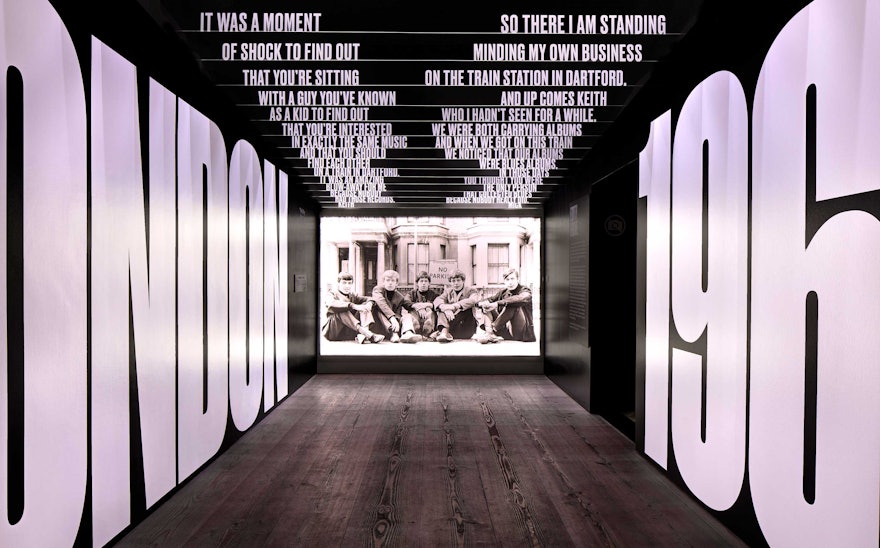This is an indoor photo of an artistic museum exhibit, possibly dedicated to historical music, particularly the Rolling Stones. The viewer looks down a hallway with walls and ceiling painted in deep black, creating a dramatic backdrop. Large white letters stretch from floor to ceiling on both walls. The left wall reads "London," but only the letters "O-N-D-O-N" are visible, while the right side is partially obscured by the image, displaying "1960" and part of another digit. The floor is wooden, with visible grain and eye-catching patterns.

As you walk down the hallway, towards the focal point at the end, words cascade from the ceiling in two columns. They narrate a significant moment: "It was a moment... so there I am standing... shocked to find out... that you're sitting with a guy you've known as a kid... interested in exactly the same music..." The text appears to recount the chance meeting of Mick Jagger and Keith Richards at a train station in Dartford, recounting the discovery of their mutual love for blues records.

The hallway culminates in a black-and-white photograph of five men sitting in front of a Victorian-style house, representing the Rolling Stones in their early years. The evocative quotes above and the historical context provided by the surroundings make this a compelling and immersive exhibit.